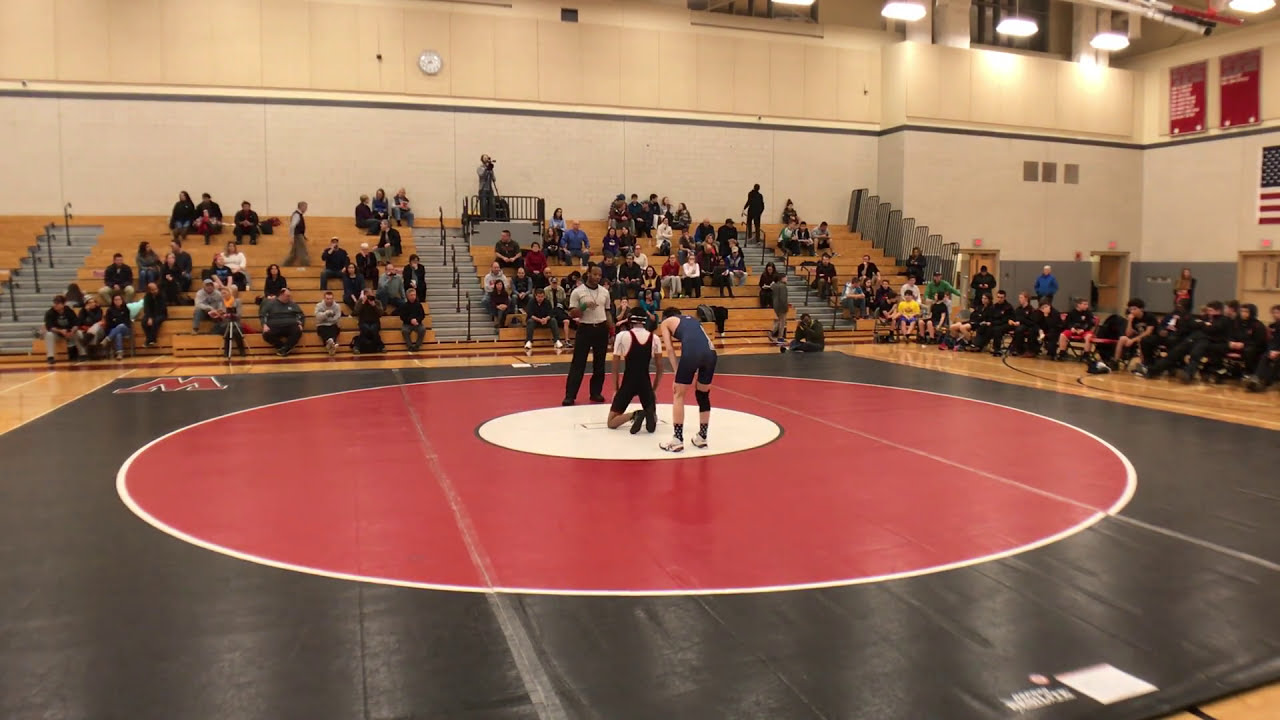This is an image from a high school or junior high school wrestling tournament, set inside a brightly lit gymnasium. The focal point is a large, square wrestling mat that dominates the gym floor. The mat is primarily black with a prominent red circle and a smaller white circle inside it. A "W" logo suggests the high school's team identity. 

Two wrestlers are positioned on the mat within the white circle: one in a blue singlet is hunched over another in a black and red singlet who is on his knees, both facing away from the camera. A referee in a white shirt and black pants stands in front of them, his right hand raised, seemingly ready to start the match.

In the background, approximately half-full bleachers stretch across the width of the image, filled with spectators. Near the mat's edge, additional chairs accommodate other team members. The gym's walls are adorned with banners showcasing state championships in various sports, an American flag, and the gym's lighting fixtures. Guardrails next to the bleachers provide safety for those stepping up. Multiple doors, including a fire exit, and ventilation systems are visible along the walls, hinting at the gym's functionality and safety measures. Overhead, there appear to be office spaces that offer a bird’s-eye view of the ongoing tournament, adding a unique and practical dimension to the gym's design. The image captures an engaging and lively atmosphere.